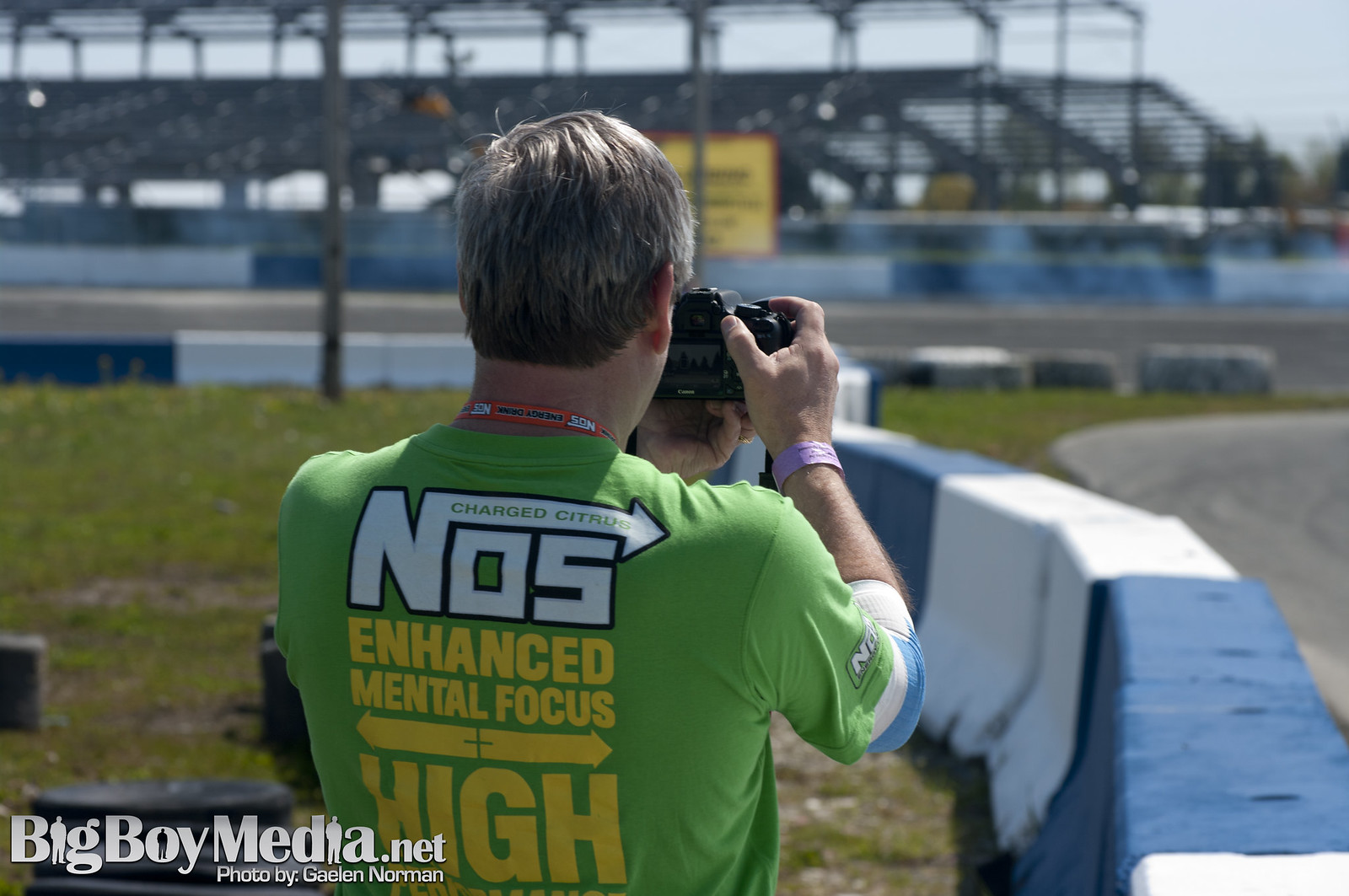In this detailed photograph by Galen Norman, we see an older white male with black and gray hair, wearing a green t-shirt that reads "CHARGE CITRUS NOS ENHANCED MENTAL FOCUS" in yellow and white lettering, along with arrows pointing in both directions and the word "HIGH." He is holding a black camera, either a Canon or Nikon, up to his face, capturing a scene at a racetrack. The man has a lanyard, likely with an ID card, around his neck and a wristband on his right wrist. The background reveals blue and white barricades along the racetrack, with spectator bleachers and stands dimly visible in the distance. The grassy area outside the track and the logo "bigboymedia.net" in the lower left corner add additional context to this motor racing event setting.